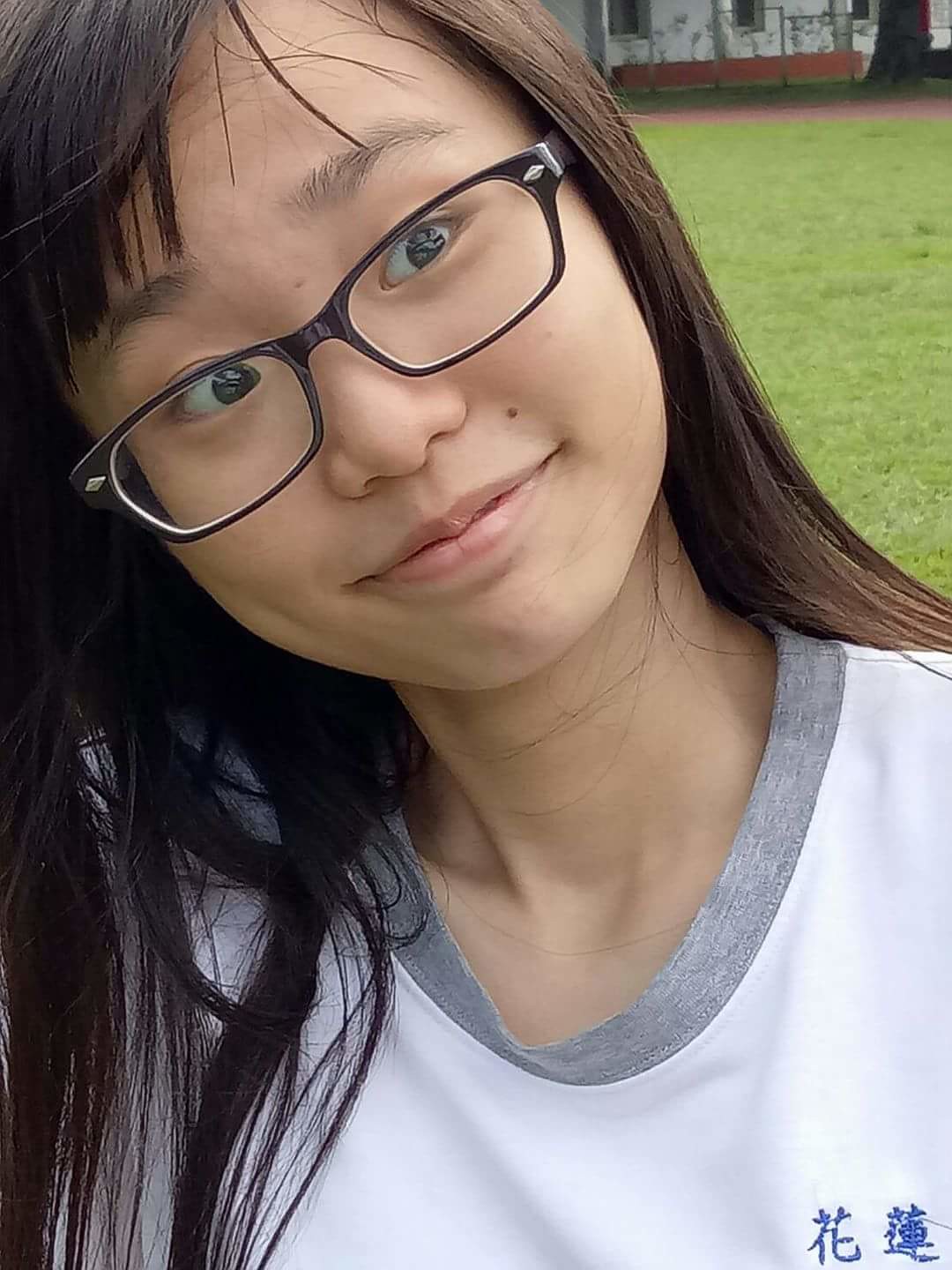The image is a candid photograph captured outdoors on a sunny day, featuring a young Asian girl, possibly aged between 16 and 20. She has long brown hair with bangs, and is wearing black-rimmed glasses over her brown eyes. Her head is tilted slightly to her right as she looks off to her left, away from the camera, while making a subtle smirk. She has a distinctive birthmark just above her upper lip. She is dressed in a white shirt with a gray collar, which features some Japanese characters in blue in the bottom right corner. The background reveals a sports field with grass, a bit of a red track, a fence, and a building with a red base. Also visible is a black sign with white and red font, although the text is unclear due to distance. The photo appears to be taken in a park or similar field area.